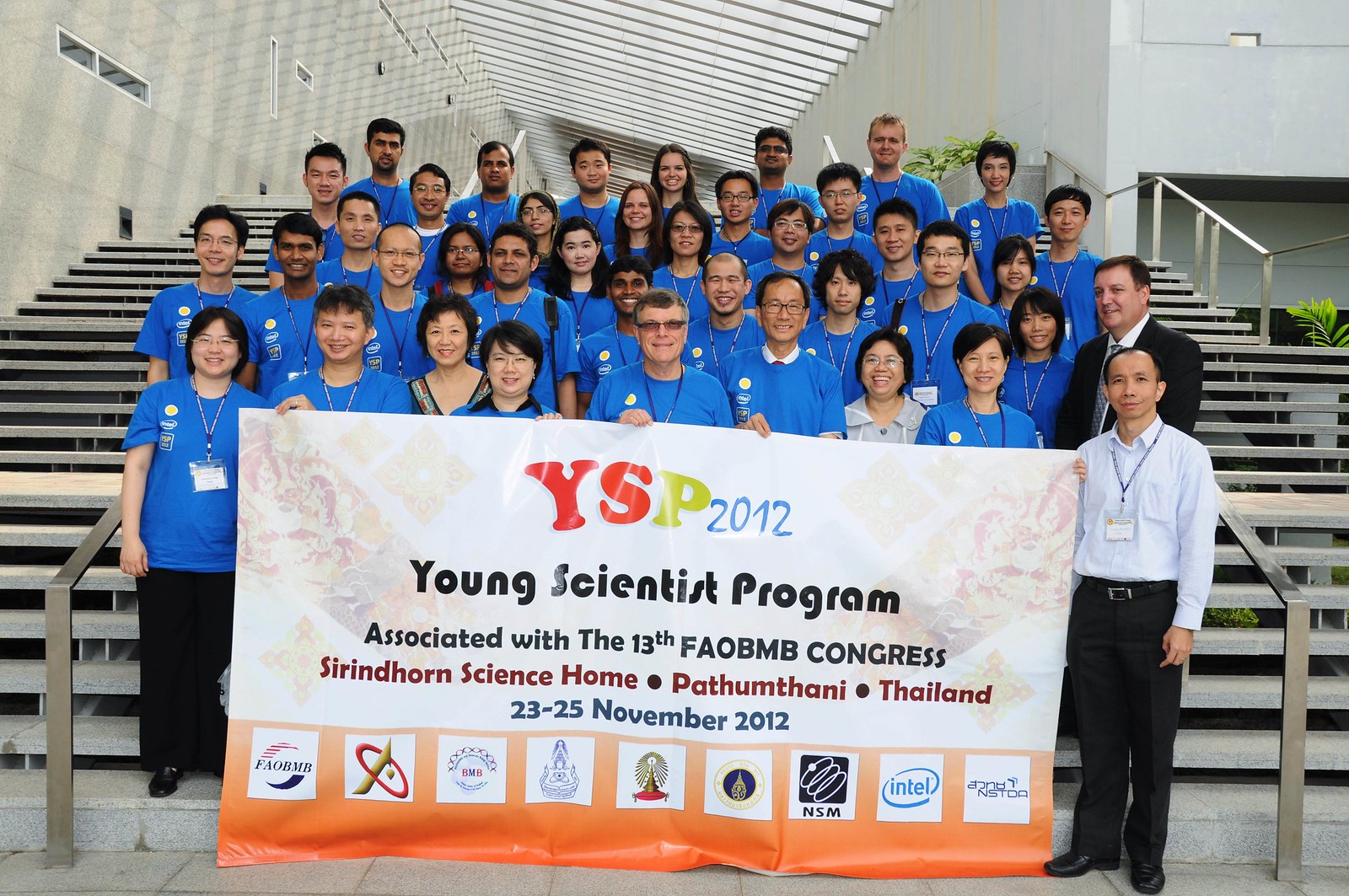In this vibrant group photo, taken on a staircase in front of an open building with a visible angled roof, around 25 individuals are gathered in six rows. Everyone in the group, a mix of men and women, is donned in blue t-shirts featuring logos on the left chest, signifying their participation in the Young Scientist Program (YSP). Prominently, two gentlemen, likely teachers or officials, stand out in the front row: one in a white business suit with a blue tie and another in a black business suit with a black tie. These two are holding up a white banner that announces "YSP 2012" in colorful text - the "Y" in red, the "S" in red, the "P" in gold, and "2012" in blue. Below, in black letters, the banner reads: "Young Scientist Program, Associated with the 13th FAO-BMB Congress, Surin Horn Science Home, Pathuthani, Thailand, 23-25 November 2012." The bottom of the banner features an orange gradient section displaying logos of nine supporting companies, emphasizing the collaborative nature of this significant scientific event.